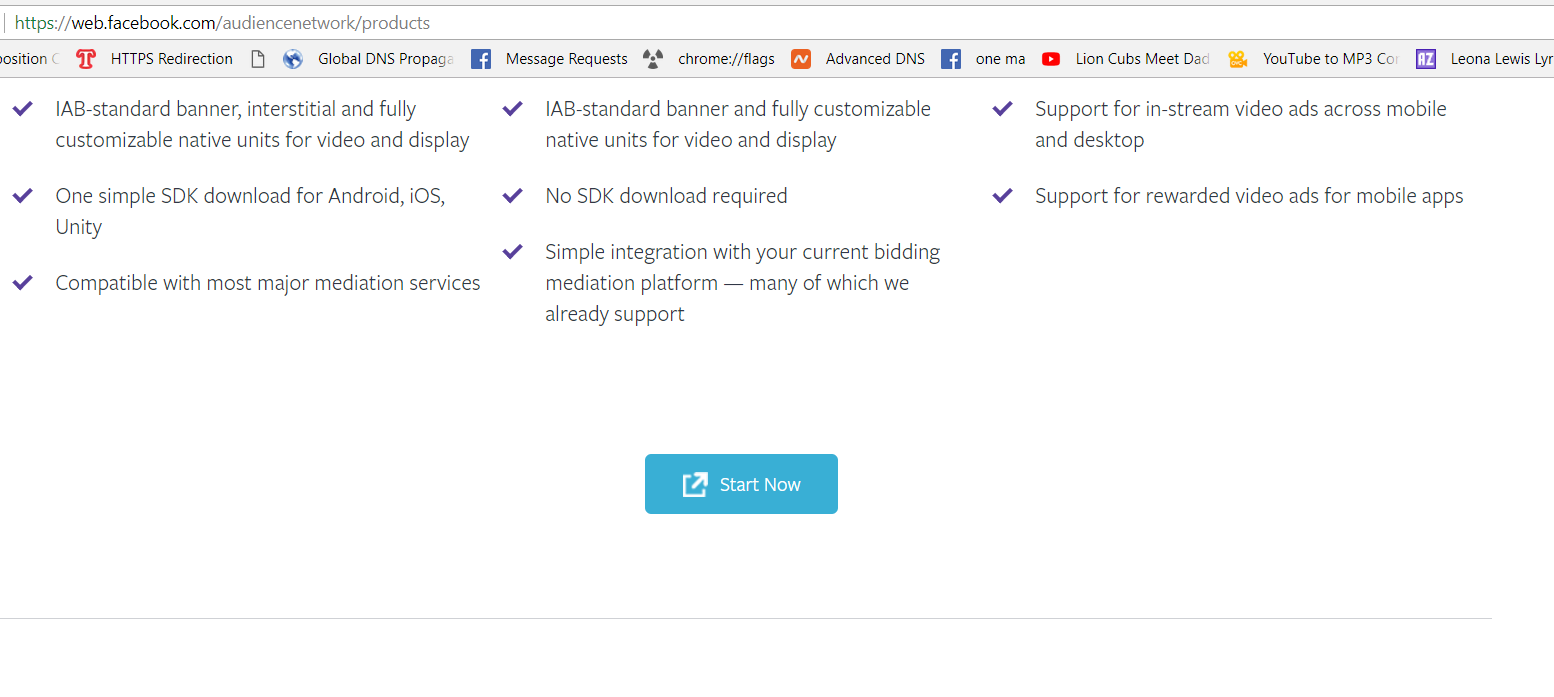This image is a partial screenshot of a web browser displaying a webpage. Although the image is cropped, the URL bar is still visible at the top, featuring a white background. The URL area shows "HTTPS" in green followed by "web.facebook.com/audience_network/products" in black text. Below the URL bar is a bookmarks bar that extends across the screen but is truncated on both sides. The visible bookmarks include partially obscured titles and icons, such as a red symbol for HTTPS redirection, a globe icon for global DNS, and several other icons that are cut off or fade out due to their length. Notable bookmarks include "Message request from Facebook," "Chrome/flags," "Advanced DNS," "1MA" with a Facebook icon, "Lion, Cubs, Me" with a YouTube video recorder icon, "YouTube 2MP3," and an AZ Lyrics website icon.

Below the bookmarks bar lies the main content of the webpage, which is set against a white background. The content is organized into three columns of text, each beginning with purple check marks on the left side. The columns appear to be part of a comparison table, possibly comparing three different pricing plans or service features, although the title of this table isn't visible due to the scroll position. 

The text in the first column reads, "IAB standard banner, interested and fully customizable native units for video and display." The second column contains similar text: "IAB standard banner and fully customizable native units for video and display." The third column states, "Support for in-stream video ads across mobile and desktop."

At the bottom center of the webpage is a blue, rounded-corner rectangle button that includes an icon denoting navigation to another website, which is depicted as a square with an arrow emerging from it. The button is labeled "Start Now."